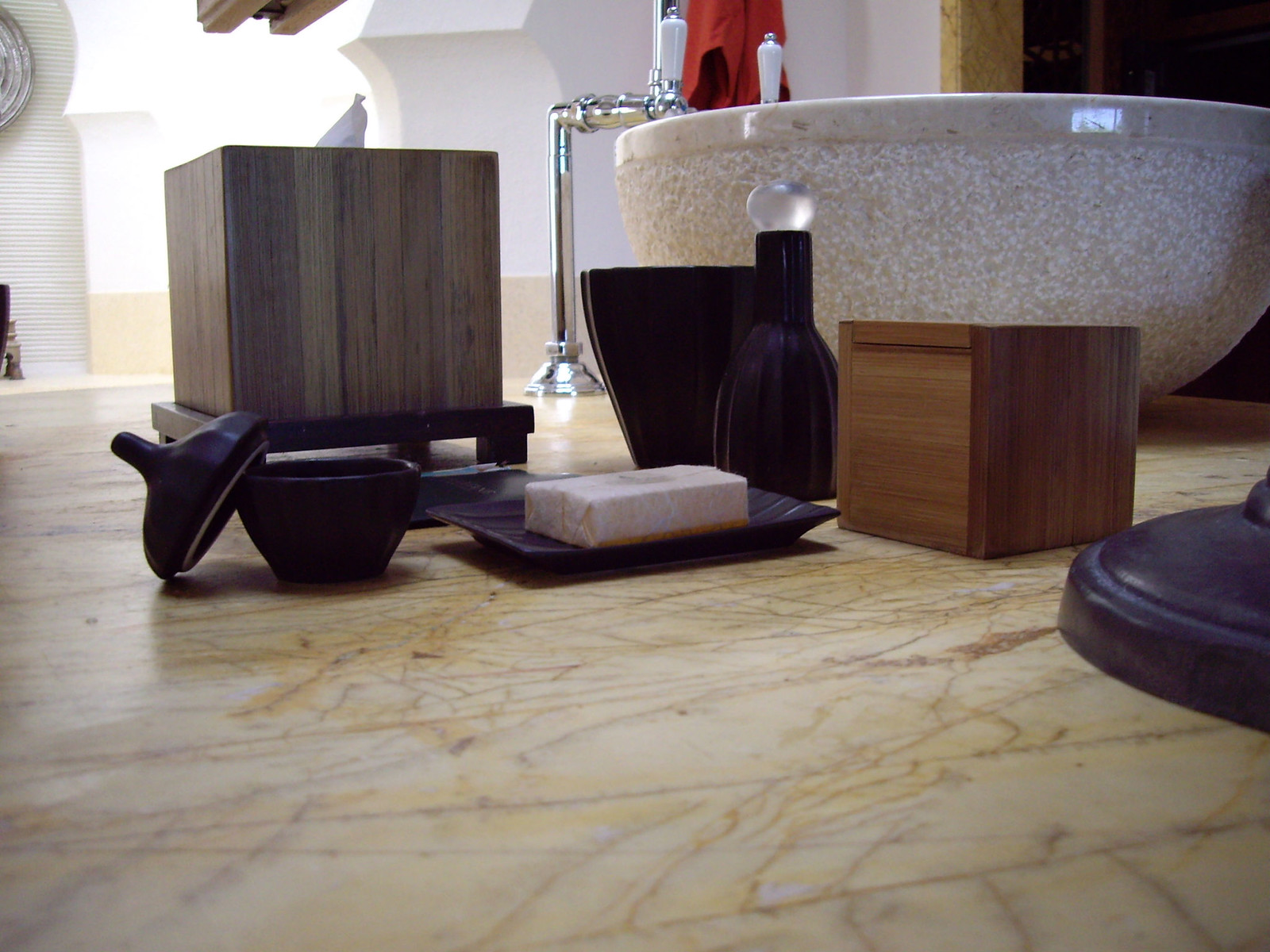This landscape-format photograph showcases a stylish bathroom countertop beside a wash basin. Captured from an angle that mimics the view if one's eyes were resting almost level with the surface, the image highlights an assortment of elegant bathroom accessories. Prominently, a bamboo-like cube container, presumably for tissues, sits in the foreground. Nearby, a larger container holds a generous stack of tissues. The eye is drawn to a sleek, black soap holder, which cradles a luxuriously wrapped bar of soap, exuding sophistication. In the distance, the round, bowl-like ceramic wash basin complements the arrangement, while a red towel hangs neatly on the wall behind, adding a pop of color to the chic setting. This meticulously arranged scene captures the essence of a high-end bathroom akin to those featured in glossy magazines.